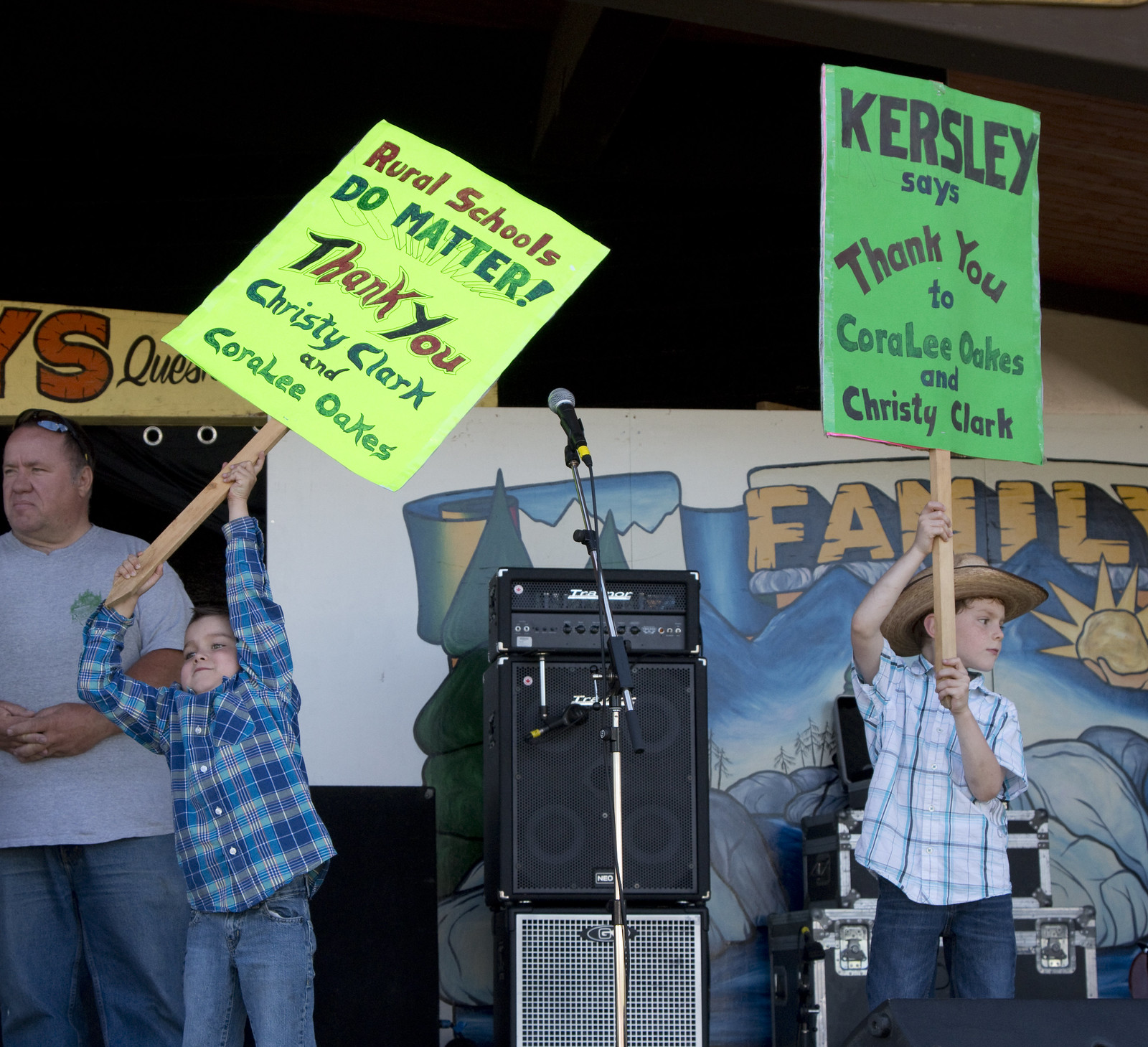In this color photograph, there is a stage set against a painted backdrop featuring a mountain landscape with a river and the Sun in the sky, with the word "Family" prominently displayed. An adult man in a t-shirt and blue jeans stands on the far left side of the stage. Next to him, two small boys are positioned near a microphone and a large speaker. Both boys are dressed in plaid shirts and blue jeans. The boy to the left, near the adult man, is holding a neon yellow picket sign that reads, "Rural Schools Do Matter. Thank you, Christy Clark and Cora Lee Oaks." The boy on the right, who is also wearing a cowboy hat, holds a green sign stating, "Cursley says thank you to Cora Lee Oaks and Christy Clark."